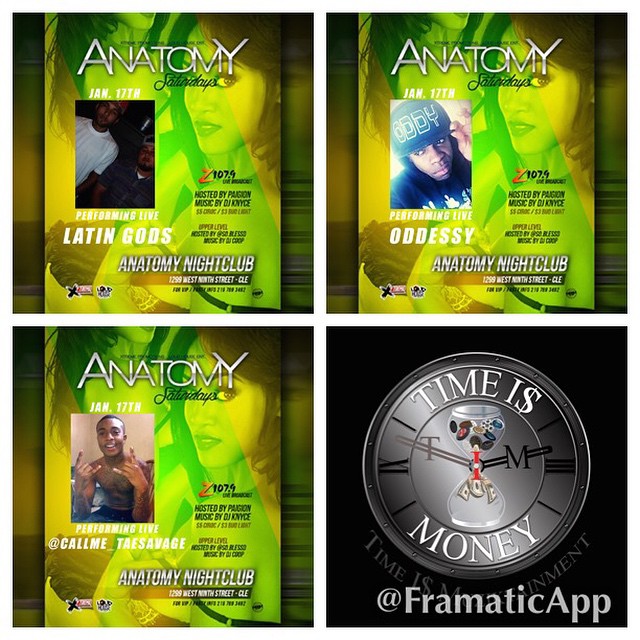The image is divided into four distinct squares, three of which prominently advertise "Anatomy Saturdays" at a nightclub, featuring live performances by different artists. The top left square announces "Performing Live: Latin Gods," while the top right highlights "Performing Live: Odyssey." The bottom left square presents "Performing Live: Call Me Trey Savage." Each of these sections has a predominantly green background with the silhouette of a woman. The shared details in all three include text stating "Anatomy Saturdays, January 15," with music hosted by Pygon and DJ Knice, price listings of $5 for rock and $3 for light, and the venue address at "Anatomy Nightclub, 1299 West 9th Street, CLE." The bottom right square deviates with a black background showcasing a clock that reads "Time is Money," alongside an hourglass logo and a reference to an "Affirmative App."